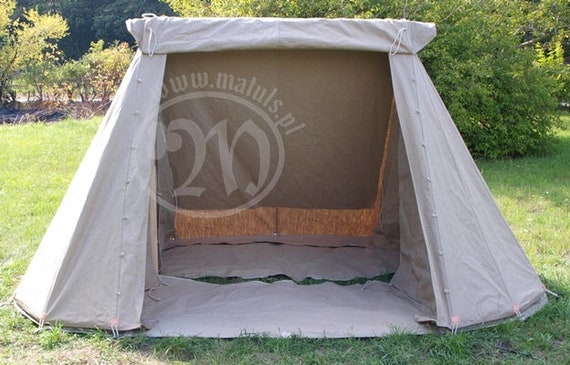The photograph captures an outdoor setting on a sunny day, featuring a gray, trapezoidal tent with almost no curves on the sides, pitched in a well-maintained, green grassy area with trees and bushes in the background. The tent is rectangular in shape, approximately 4 inches wide by 2 to 3 inches tall in the photograph. The front of the tent is open, with its flap rolled up and secured at the top, revealing an interior that appears dark, suggesting good light-blocking properties. The tent's floor is divided into segments, allowing patches of green grass to show through. Supporting the structure are white fabric and strings on the sides. Overlayed on the image is a transparent light brown circle with a stylized three-leaf clover, followed by the number 2 and possibly the letter N. Encircling the oval, the watermark reads "www.matuls.pl."